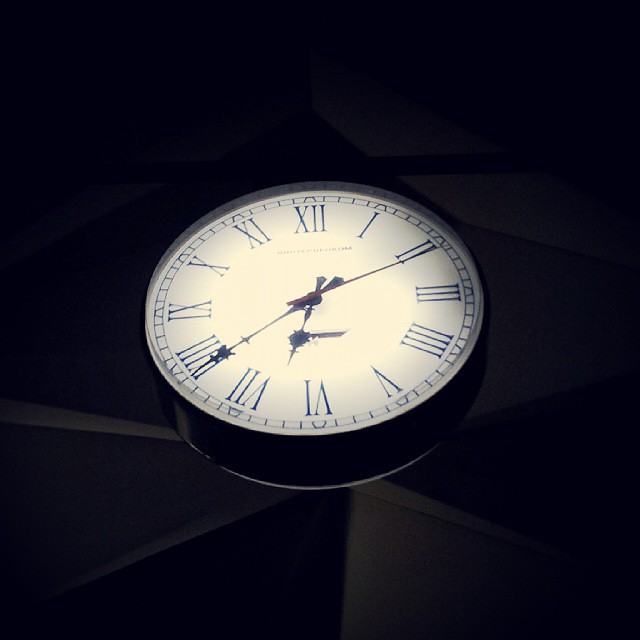This image features a classic analog clock with a white face and Roman numerals in black instead of standard numerical digits. The clock is encased in a round, sleek black rim that frames the pristine, elegant face. All three hands of the clock—the hour, minute, and second hands—are also in black, adding to the monochromatic elegance. The time displayed is 6:39, with the second hand poised near the 10 or 11 mark. Each interval between the Roman numerals is meticulously marked with smaller black lines to denote the individual minutes. The background is a gradient of black and gray shades, creating a rich, textured canvas that subtly complements the clock without drawing attention away from it. The exact nature of the backdrop remains ambiguous, adding an air of mystery to the overall composition.